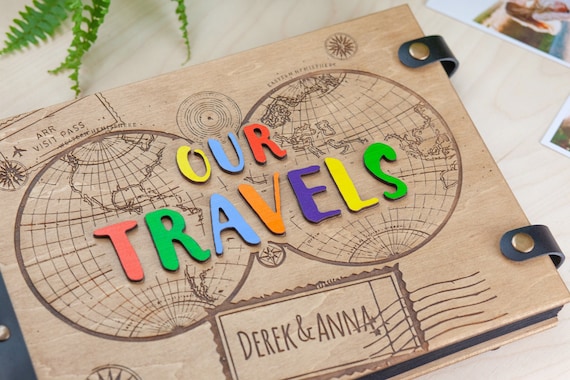This close-up photograph showcases a unique memory book or diary with a wooden cover. The center of the image focuses on the book, which is securely fastened with two black leather straps featuring silver pins, located on the right side. The cover boasts vibrant, raised lettering in various colors — "Our Travels" — with each letter in shades of yellow, blue, red, green, purple, and orange. Beneath the title, there are two engraved world maps touching each other at their edges, adding a rustic charm to the journal's appearance. A scalloped square at the bottom of the cover is inscribed with the names "Derek and Anna," while the top right corner features an engraved compass. Additionally, the upper left corner of the photograph shows the tips of fern leaves, accentuating the natural, wood-toned backdrop that complements the earthy theme of the book.